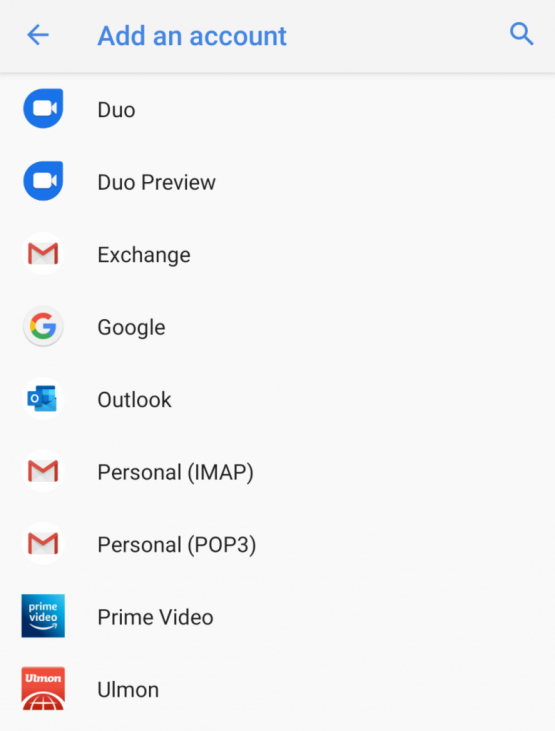The image displays a standard user interface screen featuring a light blue navigation bar at the top. In the bar, there is a small blue arrow pointing to the left, followed by the options "Add an Account" and a search icon. Below the blue bar, there is a list of account types, each indicated by a corresponding symbol. 

Aligned directly under the "A" in "Add an Account" is a sequence of account names written in black text, with each first letter capitalized: 

1. **DUO**
2. **DUO Preview Exchange**
3. **Google Outlook**
4. **Personal IMAP**
5. **Personal POP3**
6. **Prime Video**
7. **ULMON**

Notably, the word "ULMON" is highlighted in red and accompanied by a unique symbol, which consists of half an upside-down circle with a smaller circle inside it.